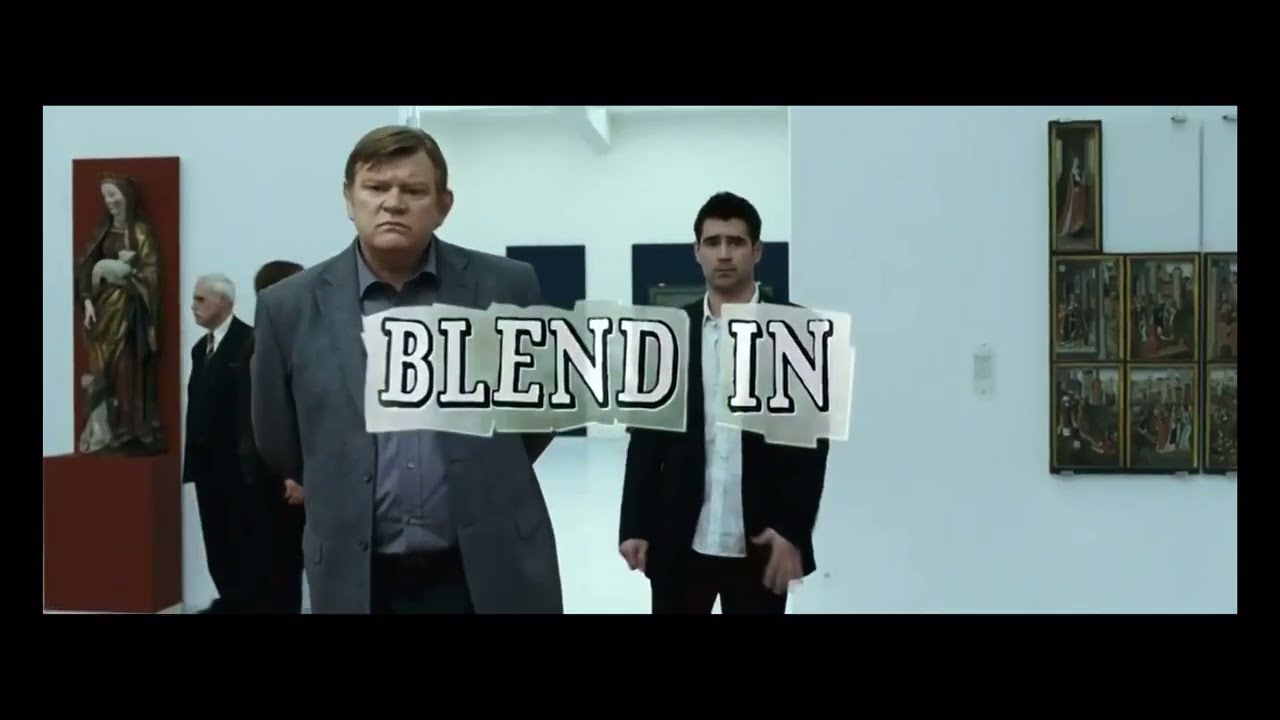In the image, there is a detailed scene that appears to be a screenshot from a movie, featuring the actor Colin Farrell. He is prominently positioned in the center, dressed in a black suit coat, black pants, and a white dress shirt. Next to him on the left is another man in a gray suit with a light gray shirt and gray pants. The two men are looking towards the camera, but not directly at it. Surrounding them is an indoor setting that resembles an art museum, characterized by white walls and various artworks.

On the right side of the image, there are several small religious paintings in gold frames hanging on the wall. On the left, there is an image of a statue of the Mother of Mary, placed on a red base with a red wall behind it. In the background, behind the man in the gray suit, there are people who appear to be security guards dressed in all-black suits. The scene has a cinematic feel, heightened by thick black lines framing the top and bottom of the image, with thinner lines on the sides.

In the center of the image, overlapping the two men, there is text in a silver font that reads "Blend In." The overall color palette includes white, black, gray, light blue, red, yellow, brown, and silver, enhancing the visual richness of the scene. The meticulous details and composition suggest that this is a dramatic and carefully crafted moment within the film or show.